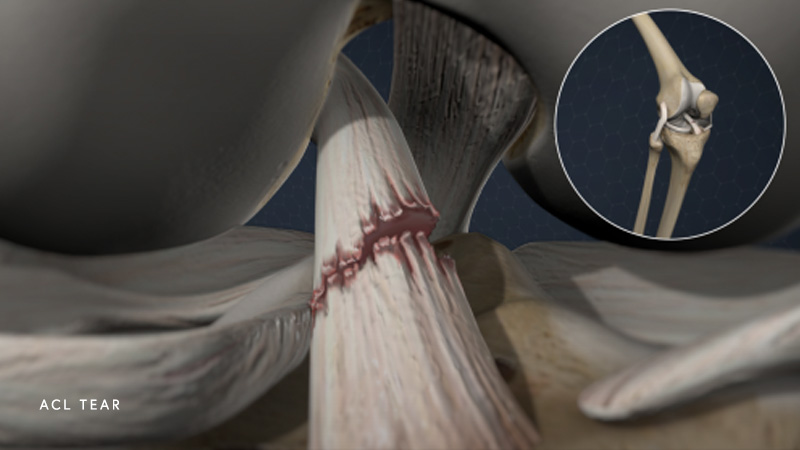This detailed caption captures various aspects from the three voice-generated inputs:

The image is a computer-generated, close-up visualization of an ACL tear in the knee. The main portion of the image highlights the exact location of the tear with enhanced color details, emphasizing red to indicate trauma. A small circular inset within the image further pinpoints the area of the tear, effectively zooming in on the involved ligament. The rendering is highly detailed; it depicts the ligament appearing as though it has been ripped in half. Accompanying this visual is the text "ACL TEAR" situated in the bottom left-hand corner in white, all-capital letters. Although the main colors are mainly whites and grays, depicting the bone and torn ligament, the red hints at the traumatic impact. This image seems ideal for educational purposes, providing a clear and precise illustration of an ACL tear in a computer-generated format rather than a real-life x-ray or photograph.